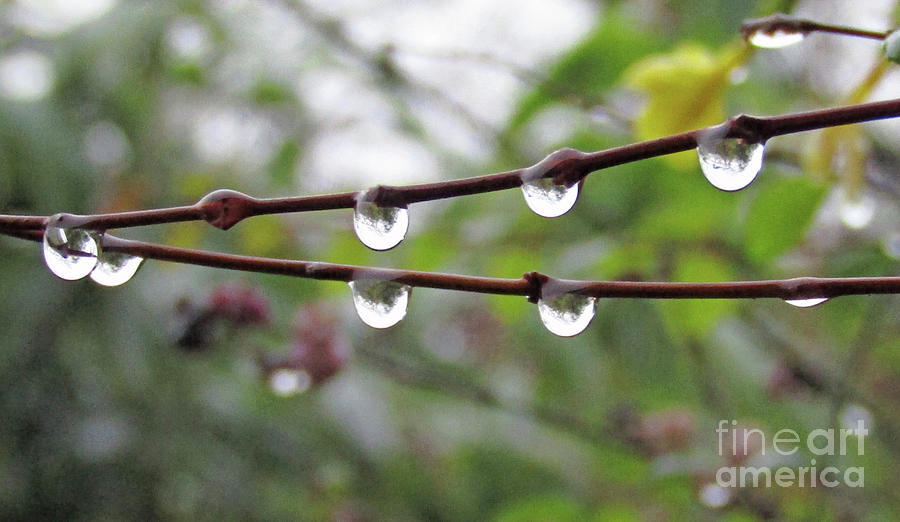This photograph captures an extreme close-up of two slender plant branches, appearing as if they are connected towards the ends before diverging and spreading out into the frame. The branches, characterized by a dark brownish-red hue and dotted with small bumps, are heavily drenched from what appears to be rain, showcasing seven fully formed water droplets poised to fall, while an eighth drop is in the process of forming. The accumulated rain imparts a sense of condensation or freezing. The blurry background hints at a densely forested area with varying shades of green and dark-colored branches. Notably, a cluster of yellow flower petals can be seen in the upper right, adding a touch of color contrast. The sky appears mostly white, and in the bottom right corner of the photograph, a transparent watermark reads "Fine Art America."